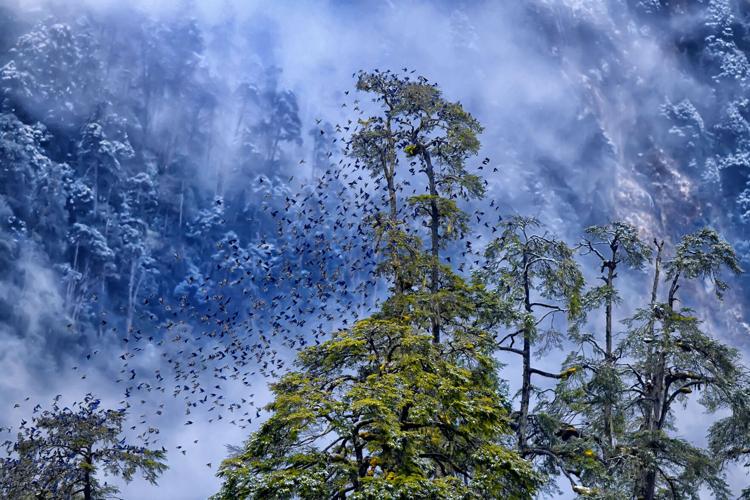This photorealistic image captures a serene early morning landscape, likely just past sunrise. The background is dominated by a soft blue hue, resembling distant, mist-covered mountains or possibly snow-capped peaks. The sky is adorned with a bluish-white tint, partially obscured by clouds and a gentle fog that rises from below, creating an ethereal atmosphere.

In the foreground, several trees stand out vividly. The central tree is lush and green, representing a typical temperate tree, though unspecified in species. To its left, a smaller tree appears darker, almost grayish, with scant green foliage. The right side of the image features a larger, more barren tree, characterized by its grayish color and sparse leaves.

Adding to the dynamic nature of the scene, a flock of hundreds of black birds is depicted in flight. These birds swoop upwards from the bottom left, heading towards the center of the image. Some birds are seen landing on the trees, while others fly away, creating a sense of movement and life amidst the tranquil setting. The interplay between the vibrant birds and the misty, clouded background highlights the contrast and depth of this captivating image.